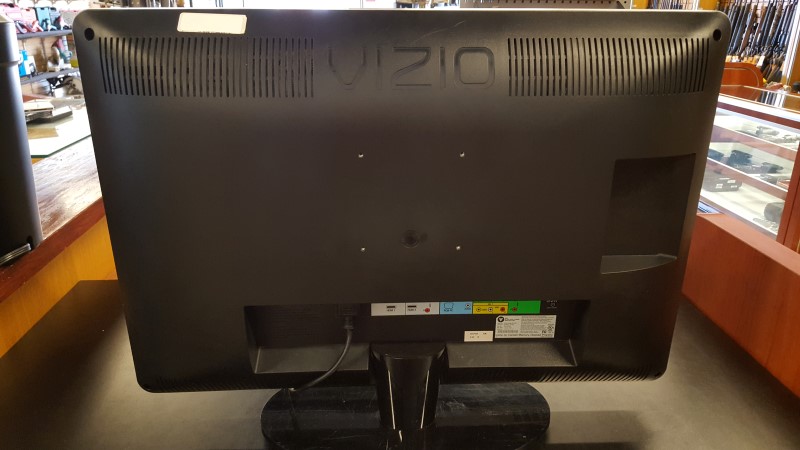The image depicts the back of a black Vizio monitor set on a glossy black desk. The monitor features horizontal grill vents at the top, the Vizio brand logo prominently displayed at the center, and four silver VESA mounting points just below it. Below the mounting points, there are various color-coded input ports, including HDMI labeled in white, and others labeled in blue, yellow, and green. A power plug is also visible extending from the monitor.

To the right of the monitor, there is a closed shelf with a brown frame and clear glass window, showcasing an array of items for sale, including men's ties hanging in the background. On the left side, there is an open shelf displaying different colorful objects in shades of pink, blue, and gray. The setting appears to be inside a store, likely a pawn shop, given the assortment of items and knick-knacks visible throughout the scene.